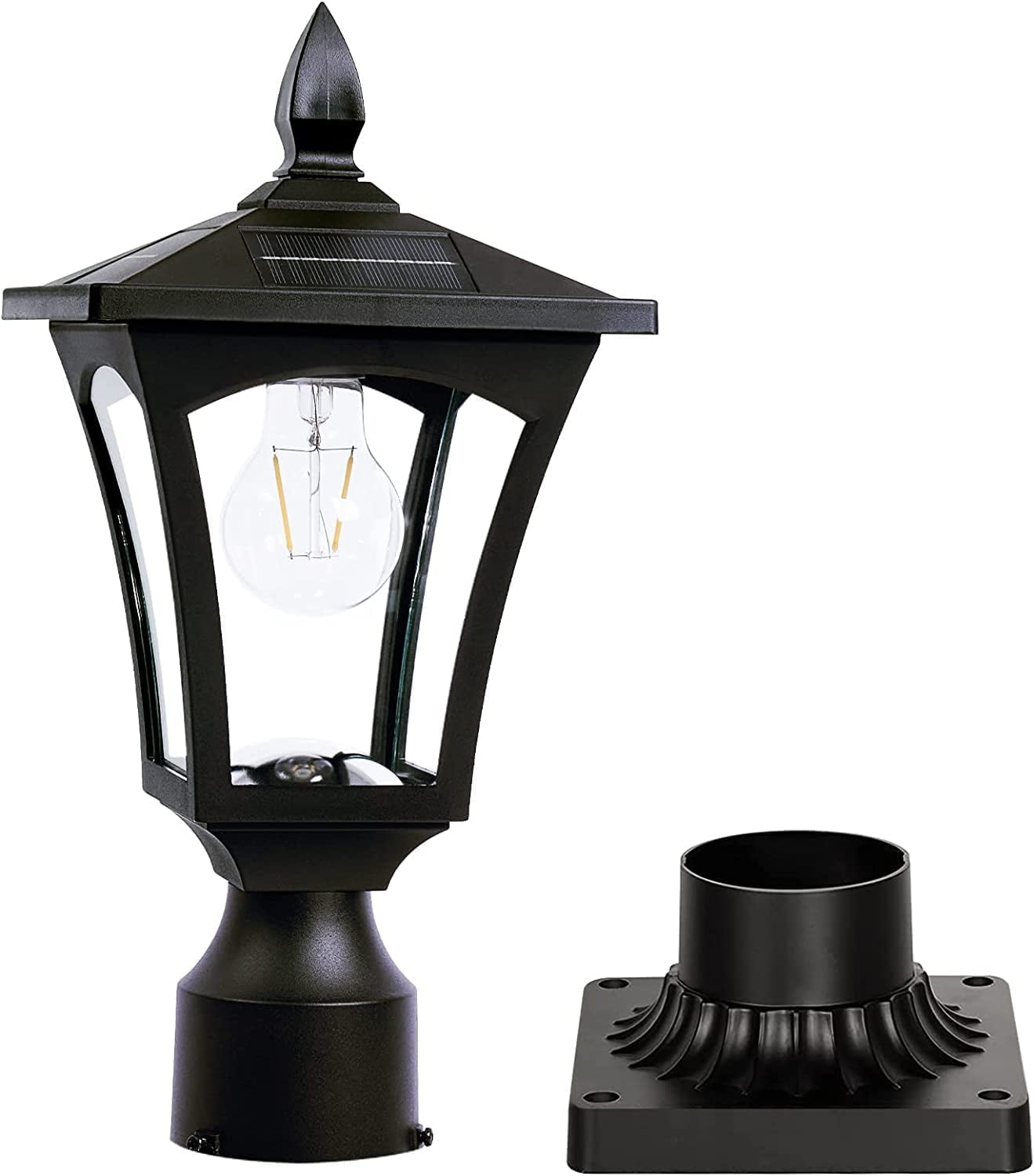This image captures an intricately designed black metal lamp with distinct parts reminiscent of old oil lamps. The lamp, heavy and rich in ironwork, is separated into an upper section housing a clear light bulb with visible filaments and a lower section which serves as the sturdy base. The upper part, shaped like a traditional lamppost with a knob on top, can be detached and reattached to the main base. This base is a square platform featuring a cylinder with gradual grooves leading to the four-cornered mounting holes, allowing for secure installation. A secondary object is present, possibly an alternative mounting option, showcasing a black matte rectangular box with similar mounting holes. This lamp, with its vintage aesthetic and potential outdoor applications, combines historical charm with functional design.